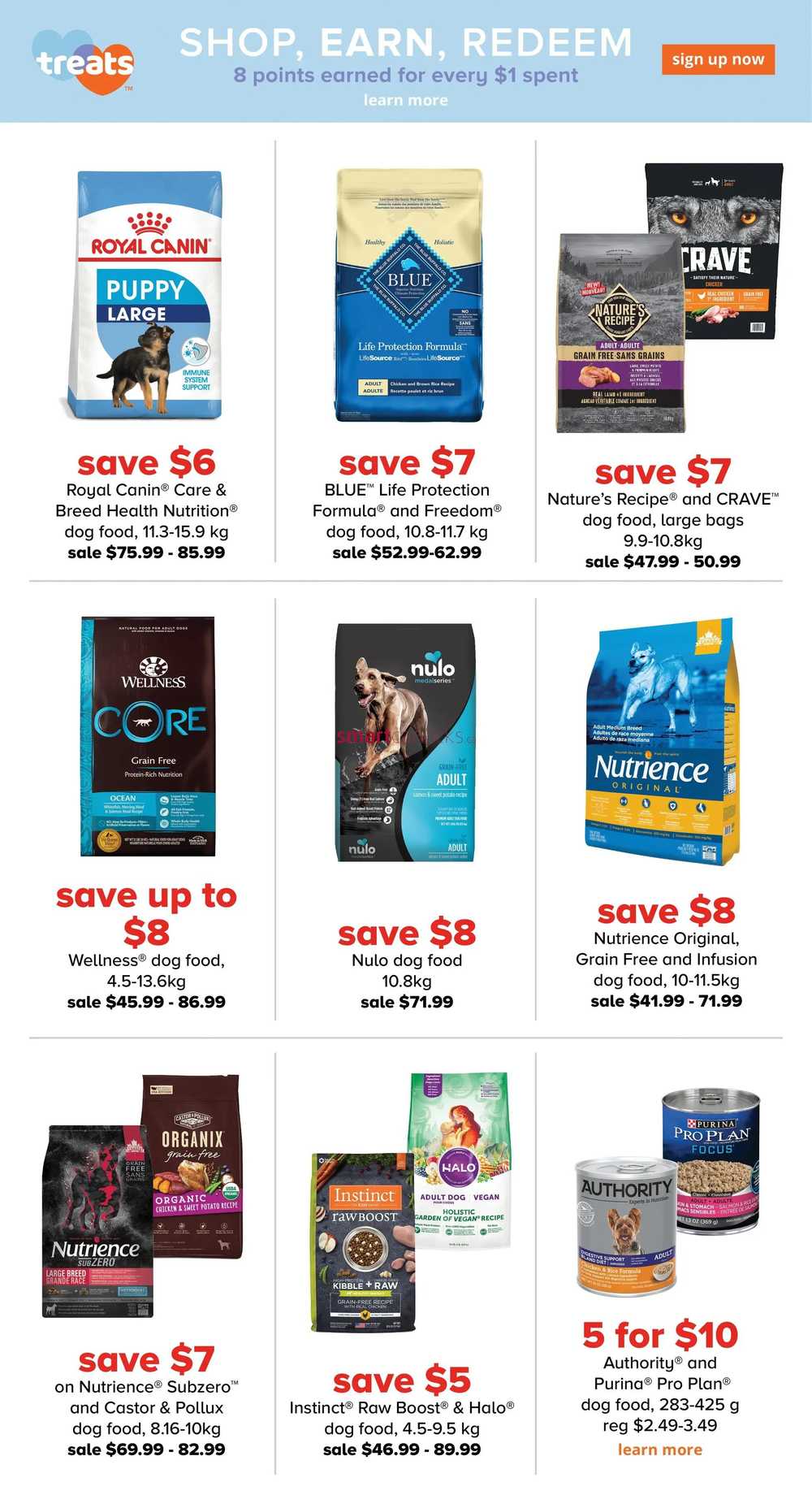The image displays a promotional section for a canine food website, laid out in a 3x3 grid format featuring various dog food products and their discounts. Here are the details in each position:

- **Top-Left:** "K9 Puppy Large" dog food with a discount of $6 displayed. The sale price range is from $75.99 to $85.99.  
- **Top-Middle:** A blue-labeled dog food with "Save $7" in red text. The sale prices range from $52.99 to $62.99.
- **Top-Right:** Two bags of dog food titled "Crave" and "Nature's Recipe." Both qualify for a $7 discount. The sale price ranges from $47.99 to $50.99.
  
- **Middle-Left:** Dog food marked with "Save $8", discounted price ranging from $45.99 to $86.99.
- **Middle:** A blue-labeled product with "Save $8". The sale price is $71.99.
- **Middle-Right:** "Nutrients" dog food marked with "Save $8", prices ranging from $41.99 to $71.99.
  
- **Bottom-Left:** Two bags, "Nutrients" and "Organics," both labeled with "Save $7". The sale pricing ranges from $69.99 to $82.99.
- **Bottom-Middle:** "Instinct" and "Hot and Hallow" dog food, both marked with "Save $5". The sale price ranges from $46.99 to $89.99.
- **Bottom-Right:** "Authority Pro Plan" canned dog food, available at five cans for $10, without additional bold price text.

Each product box includes thin black text detailing the item description, with bold text displaying the final discounted prices.